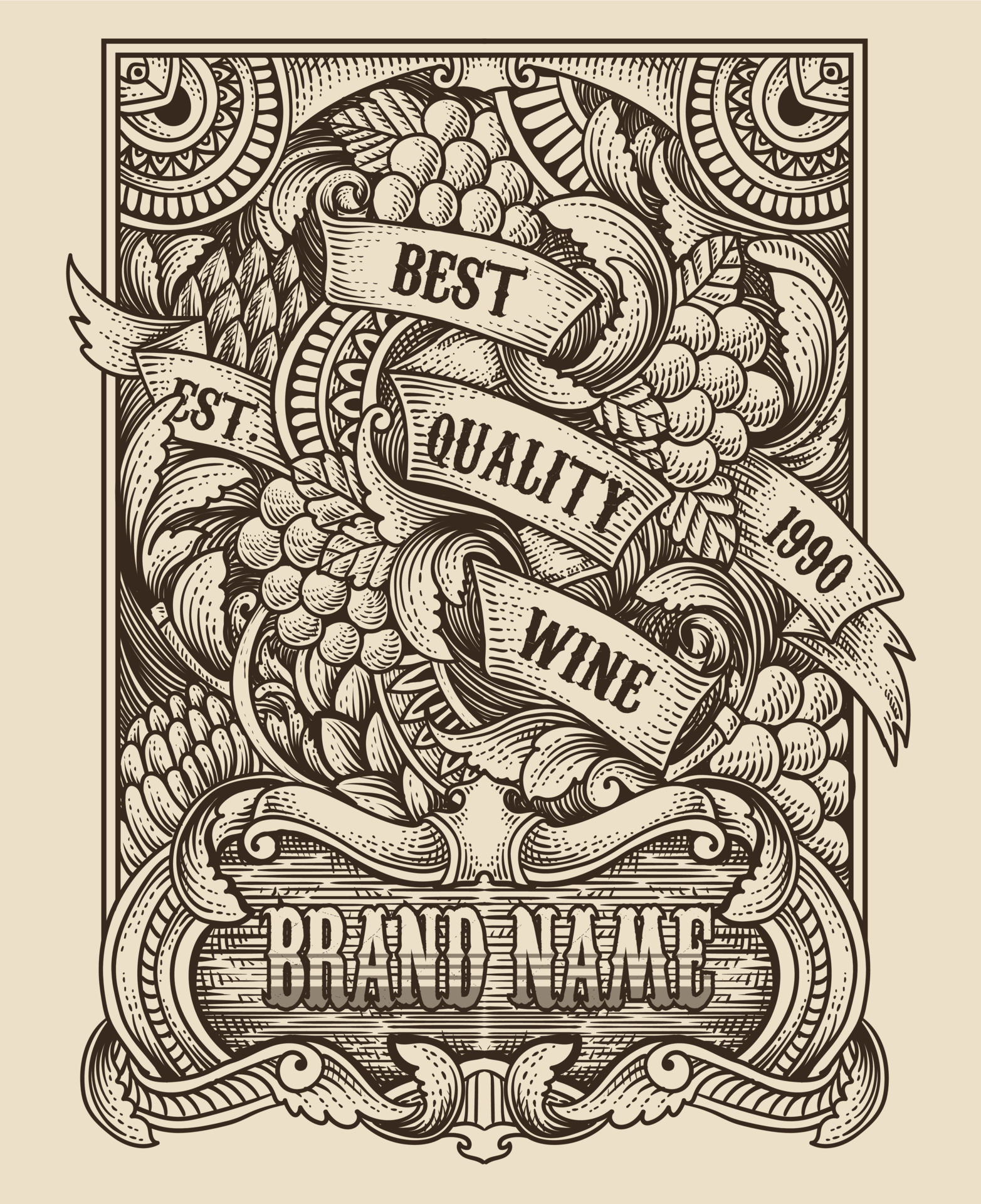This detailed black ink drawing graphic design features a cream, off-white background. The busy, squarish rectangular poster is adorned with intricate scroll work, ribbons, and decorative elements that evoke a vintage feel. At the top of the design, a ribbon emblazoned with the words "Best Quality Wine" runs through the center, with the words stacked vertically: "Best" at the top, "Quality" in the middle, and "Wine" at the bottom. The word “EST.” is placed on the left side of the ribbon, while “1990” is on the right, indicating the establishment year.

The design is further embellished with detailed drawings of grapes and leaves, adding to its ornate, classical appearance. Below the main ribbon, at the bottom of the poster, there is an open space for customization. This space, framed by elaborate scrollwork, features the placeholder text "Brand Name" in large, hollowed-out letters, indicating where a business name could be prominently displayed.

Overall, the graphic is richly detailed and ideal for a customizable wine brand logo, providing a sophisticated, elegant depiction suggestive of high-quality, established heritage.